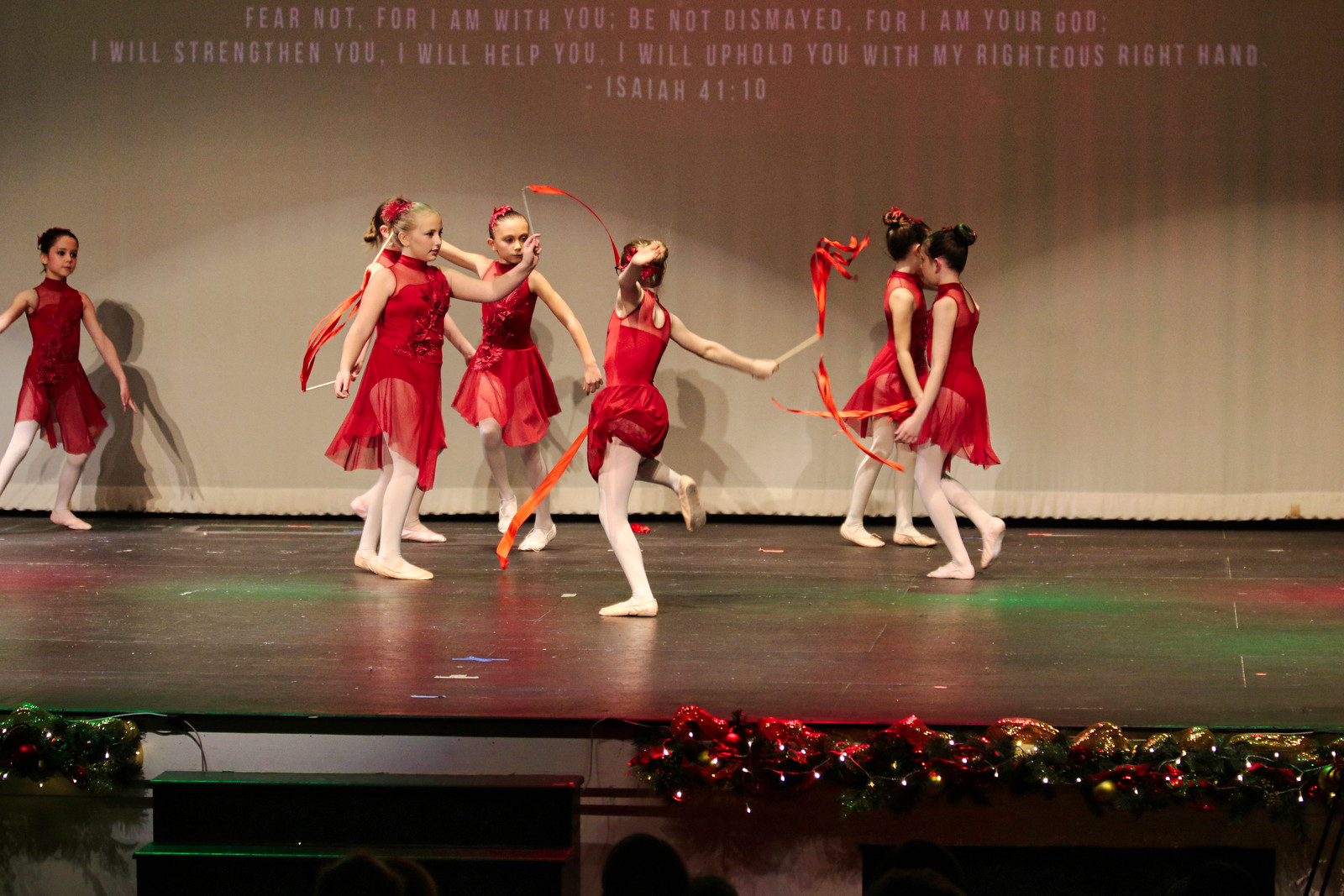The photograph showcases a vibrant dance recital with six young girls center stage and a seventh girl to the left. All dressed in red sleeveless dresses with sheer skirts, white tights, and off-white ballet slippers, these girls perform an engaging flag dance, twirling red ribbons gracefully. The stage, adorned with festive green garlands interwoven with twinkling Christmas lights, features a backdrop of a large cream curtain with a projected Bible verse: "Fear not, for I am with you. Be not dismayed, for I am your God. I will strengthen you, I will help you, I will uphold you with my righteous right hand. Isaiah 41:10." The verse is displayed in white text, adding a serene and inspirational touch. The stage itself is black, illuminated by green and red lights cast from the ceiling. Hints of the audience peek from the bottom of the frame, emphasizing the communal and celebratory atmosphere of the event, while black steps are visible on the lower left, leading to the stage.